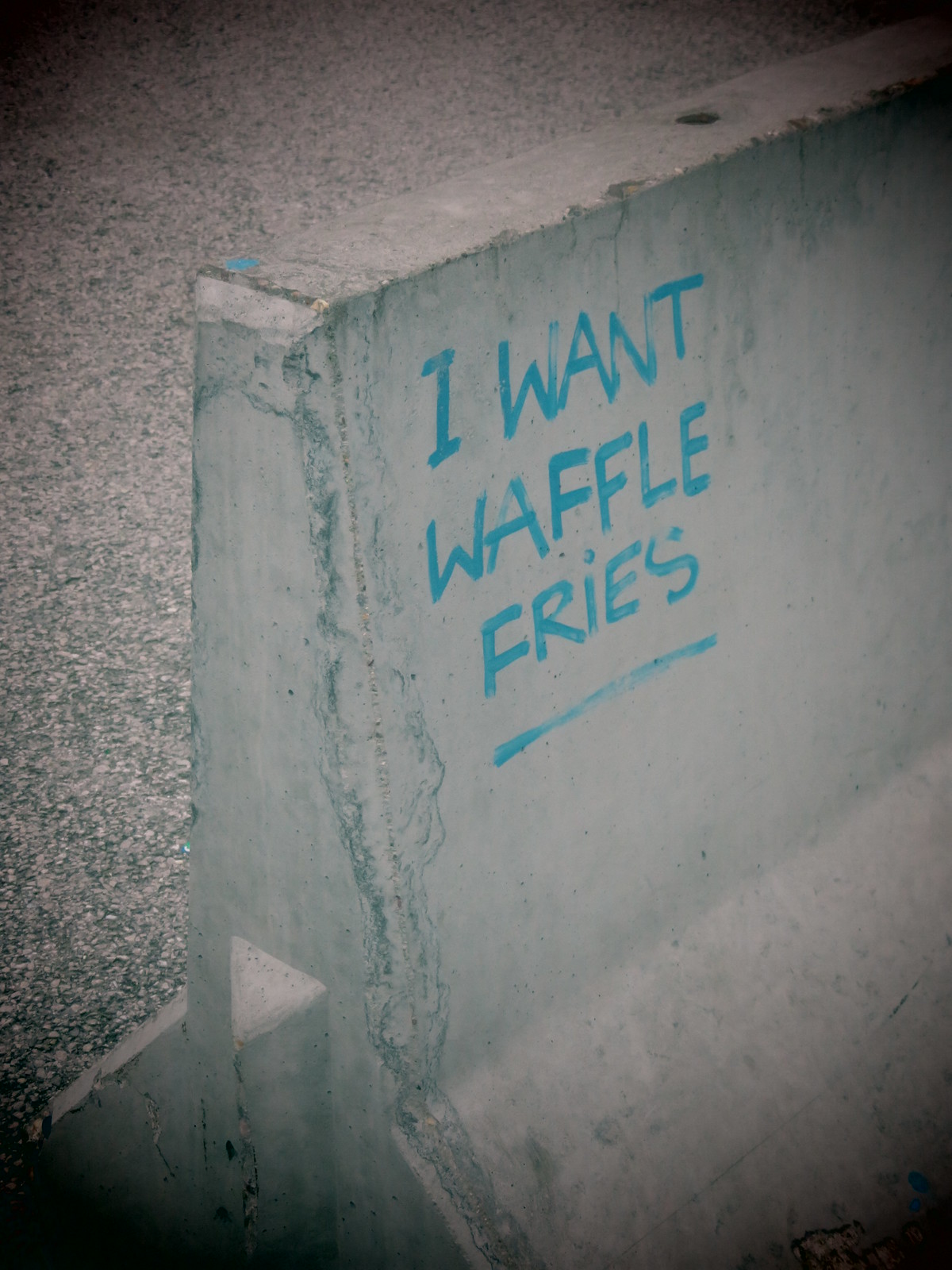The photograph, presented in a rectangular shape that is taller than it is wide, features graffiti on a weathered concrete wall. The corners of the image are darkened to black, with a light blue overlay or filter effect enhancing the overall view. The graffiti, written in blue magic marker or paint, says "I want waffle fries" with "fries" underlined. This inscription is located on a concrete border, often seen on streets to prevent cars from passing through certain areas. The concrete wall is quite beat up, showing chips on the top and sides, along with discoloration likely due to rain and weather conditions. The gravel on the sidewalk, made of black, red, and tan stones, rests over an asphalt base. In the top left corner of the photo, the very base of a streetlight is visible. The concrete wall itself features a flat, narrow top that transitions into a broader side, flaring outward at the bottom, forming a triangular shape on both the left and right sides.